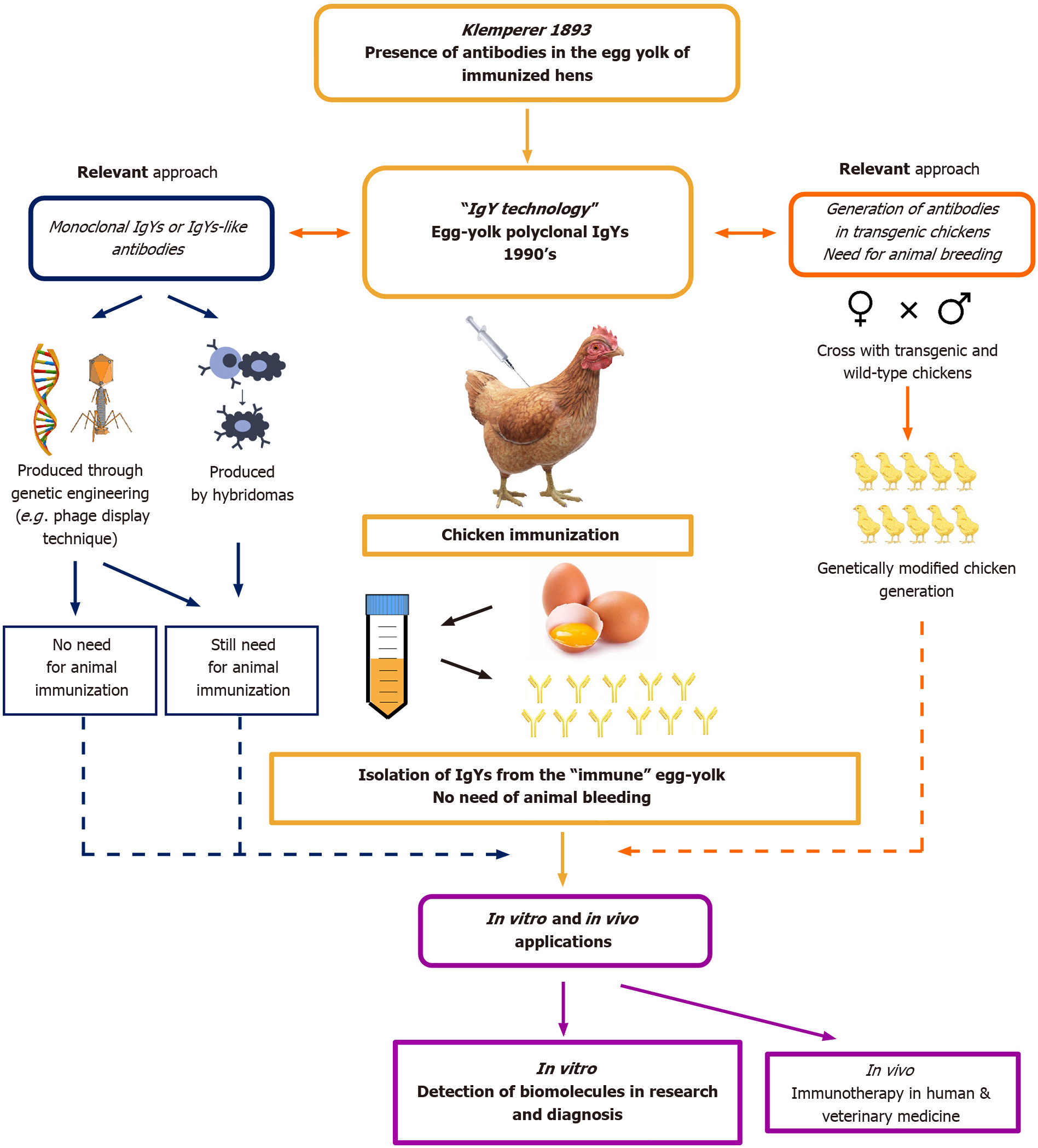The image features a white background with multiple elements arranged to convey the historical and scientific development of IGY technology. At the top, the text "Klemperer 1893" signifies the year when the presence of antibodies in the egg yolk of immunized hens was first observed. Below this, "IGY technology" is referenced, which pertains to the extraction of immune antibodies (polyclonal IGYs) from egg yolks, a significant breakthrough in the 1990s.

A chicken is prominently displayed to symbolize the role of hens in this innovative process of antibody production. Surrounding the chicken are several brown eggs, one of which is cracked open to reveal a blue, white, and brown tube, marked with "YYY" symbols, representing the isolation of IGYs from the egg yolk. This method eliminates the need for animal bleeding.

Additional text on the image highlights that the IGYs are produced through genetic engineering, with a specific approach involving transgenic and wild-type chickens. Relevant scientific applications are indicated, covering both in vitro (laboratory) and in vivo (live organism) settings.

On the right side of the image, captions point to the applications of this technology in immunotherapy for both human and veterinary medicine, showcasing its cross-disciplinary relevance and potential for advancing health treatments.